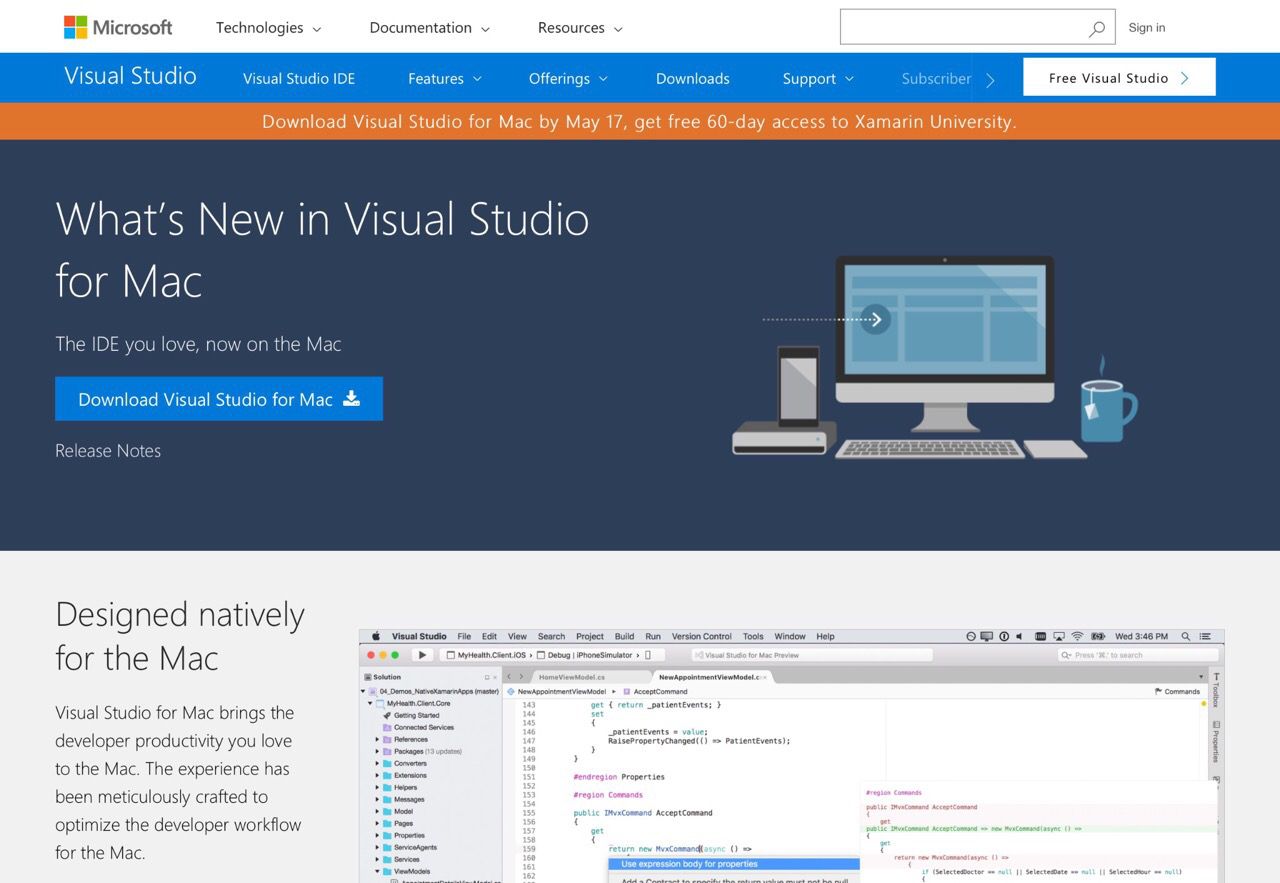This image is a detailed screenshot of the Microsoft Visual Studio website, specifically advertising its availability for Mac computers. At the top of the page, the header features the Microsoft logo on the left, followed by the word "Microsoft." To the right of the logo is a navigation menu that begins with "Technologies," "Documentation," and "Resources," each with dropdown menus. Moving further right, there is a search bar outlined in gray with a white background and a search icon. Positioned to the right of the search bar is a "Sign In" link.

Below the header, there is a prominent blue bar with the text "Visual Studio" in white on the left. This bar contains a menu starting with "Visual Studio IDE," followed by "Features," "Offerings," "Download," "Support," and "Subscriber," each accompanied by dropdown menus where applicable. On the far right of this blue bar is a white button with black text that reads "Free Visual Studio," accompanied by a greater-than symbol (>).

The next section features an orange bar with centered white text that reads, "Download Visual Studio for Mac by May 17th. Get free 60-day access to Xamarin University."

Beneath the orange bar, the hero section showcases "What's New in Visual Studio for Mac" as the largest text on the page, positioned on the left in white text. Below this headline is the subtext, "The IDE you love now on the Mac," followed by a button labeled "Download Visual Studio for Mac." Additionally, there is a link labeled "Release Notes" positioned further down. On the right side of this section is an illustration of a Mac desktop computer, set against a dark blue background.

The main content body follows, set against a light gray background. The left side features the heading "Designed Natively for Mac" in large black letters, though smaller than the previous headlines. Underneath, there is descriptive paragraph text explaining that "Visual Studio for Mac brings the developer productivity you love to the Mac. The experience has been meticulously crafted to optimize developer workflow for the Mac." On the right side is a partial image of the Visual Studio for Mac interface on a Mac UI, displaying program elements like buttons, code sections, and tabs. The image cuts off partially, leaving it unclear whether more content exists below.